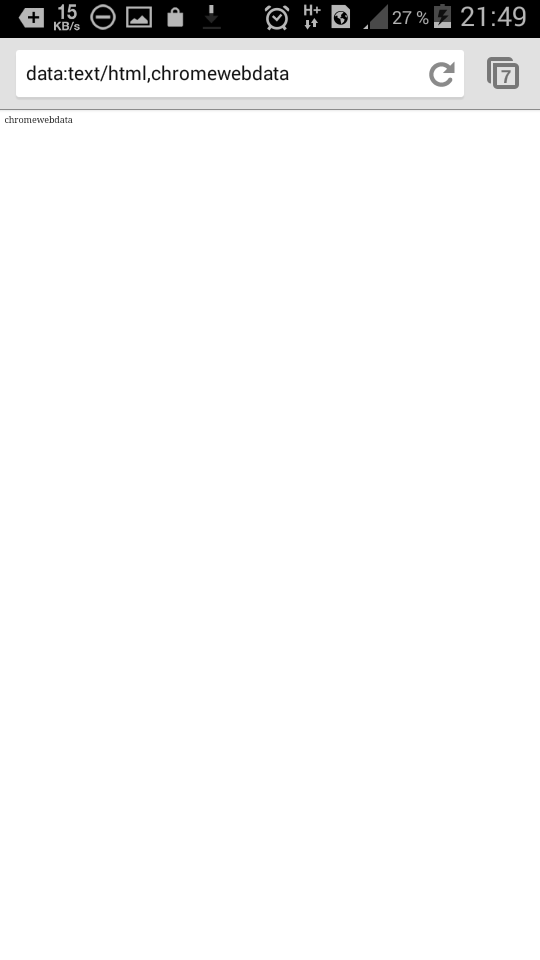The image captures a screenshot of a mobile website displaying minimal content. The phone's top status bar is visible, showing the time as 9:49 PM (21:49). The battery icon, which is gray with a black lightning bolt, indicates that the phone is charging, while the battery level is currently at 27%. The Wi-Fi connectivity appears poor, as evidenced by the single bar shown next to the battery indicator.

On the screen, the webpage content is limited to a small black text snippet at the top left corner, which reads "Chrome web data." The URL displayed is "data:text/html,Chrome web data." It's indicative of a page where an error or a blank data page is being displayed rather than actual website content. Additionally, the presence of a number "7" next to a tab icon suggests that the user has seven tabs open in their mobile browser.